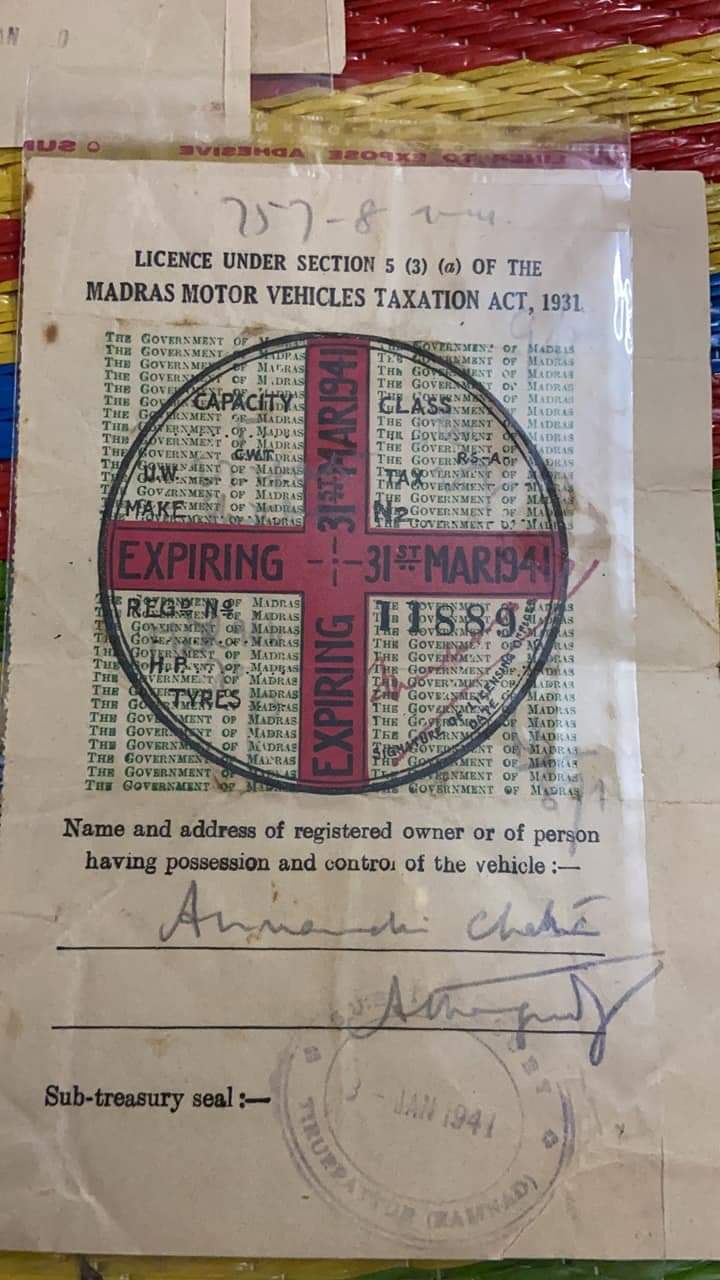This image depicts an aged and weathered piece of paper carefully preserved against a wicker background that features diagonal stripes of red, yellow, and blue. The paper, showing signs of wear such as folds and stains, is part of the "license under section 5 3a of the Madras Motor Vehicles Taxation Act, 1931." At the top, handwritten numbers "757-8" are visible, followed by the legal text. Below, there's a creative logo consisting of a red cross within a black circle, superimposed over a square filled with numbers. The words "expiring 31 March 1941" appear twice, aligned with the crossbar of the red cross. Further down, the document includes fields marked for "name and address of registered owner, or of person having possession and control of the vehicle," with illegible signatures and a notary stamp dated January 1941. The preservation efforts suggest the delicate condition of the document, emphasizing its historical significance.